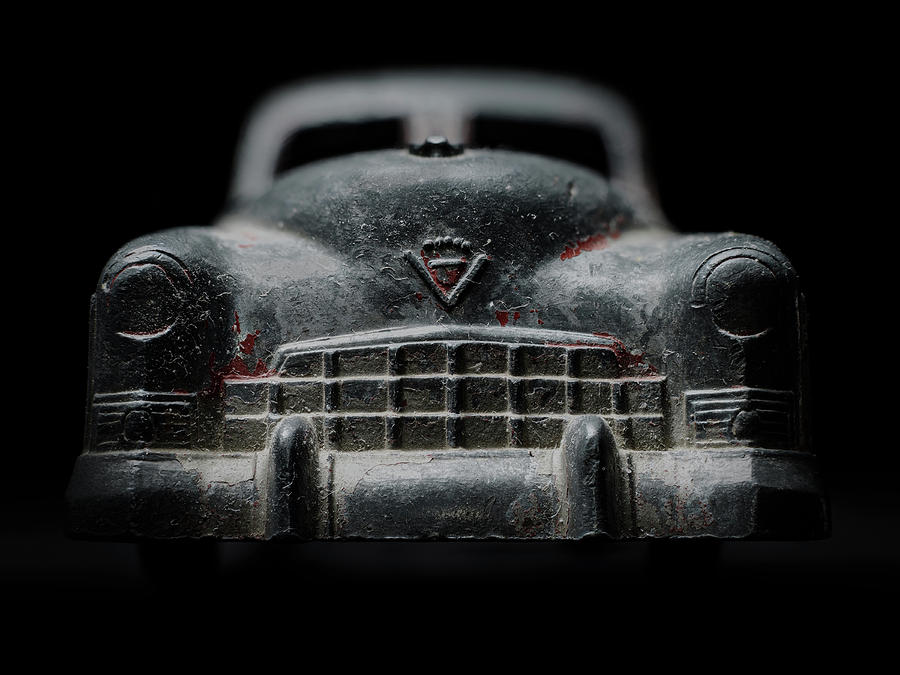The image depicts a detailed close-up of a model car designed in the style of the 1930s to 1950s roadsters. The car’s body, made of die-cast aluminum, shows significant wear with mostly silver metal exposed, but remnants of red paint still evident in streaks along its surface. The photograph, taken from a low angle, highlights the car’s distinctive V-shaped logo on the solid metal hood, intricate grille, and engraved headlight circles. A single strong light source from the front dramatically illuminates the model, casting pronounced shadows around its edges. The backdrop is entirely black, creating the effect that the model is floating in a void, further emphasizing the car’s classic rounded contours and the meticulous craftsmanship of the toy.